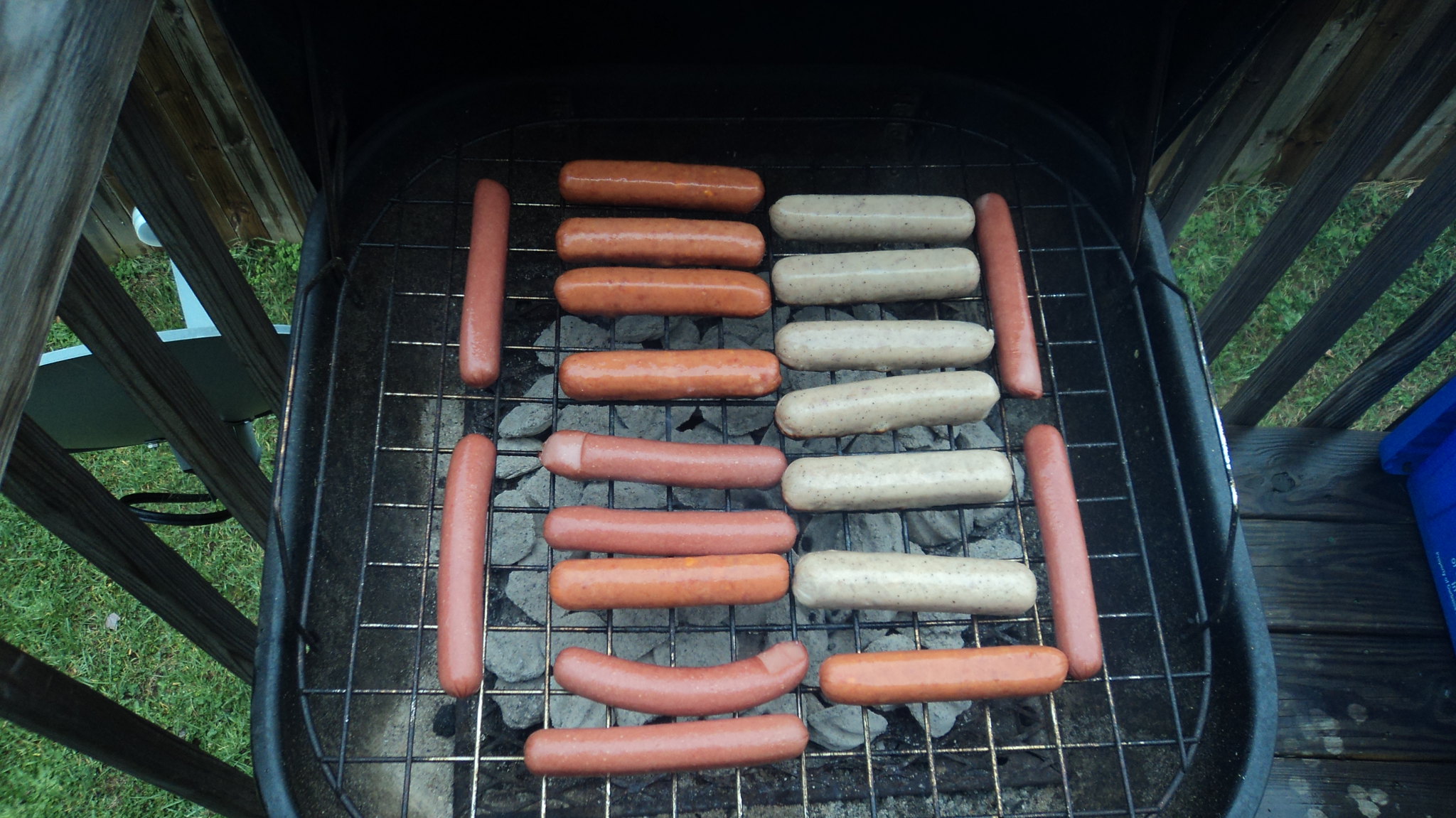In this overhead photograph, a series of hot dogs and large sausages are arranged on a black grill, situated on a wooden balcony. The perspective is from above, showcasing two vertical rows and several horizontal rows of hot dogs and sausages positioned uniformly on the grill's lined surface, ready for cooking. The hot dogs vary in color, with many being light brown, a few orangish brown, and some appearing gray on the right-hand side. The grill is prepared with fuel and charcoal, although it hasn't been lit yet.

The surrounding environment includes a gray, wooden-style flooring at the bottom right and a wooden railing with spindles on the left and top right. Small patches of grass can be seen through the railing. Additionally, a hint of a blue object is visible on the right-hand side of the image. The area is clearly higher than the ground below, indicating the grill is on a raised wooden porch or balcony.